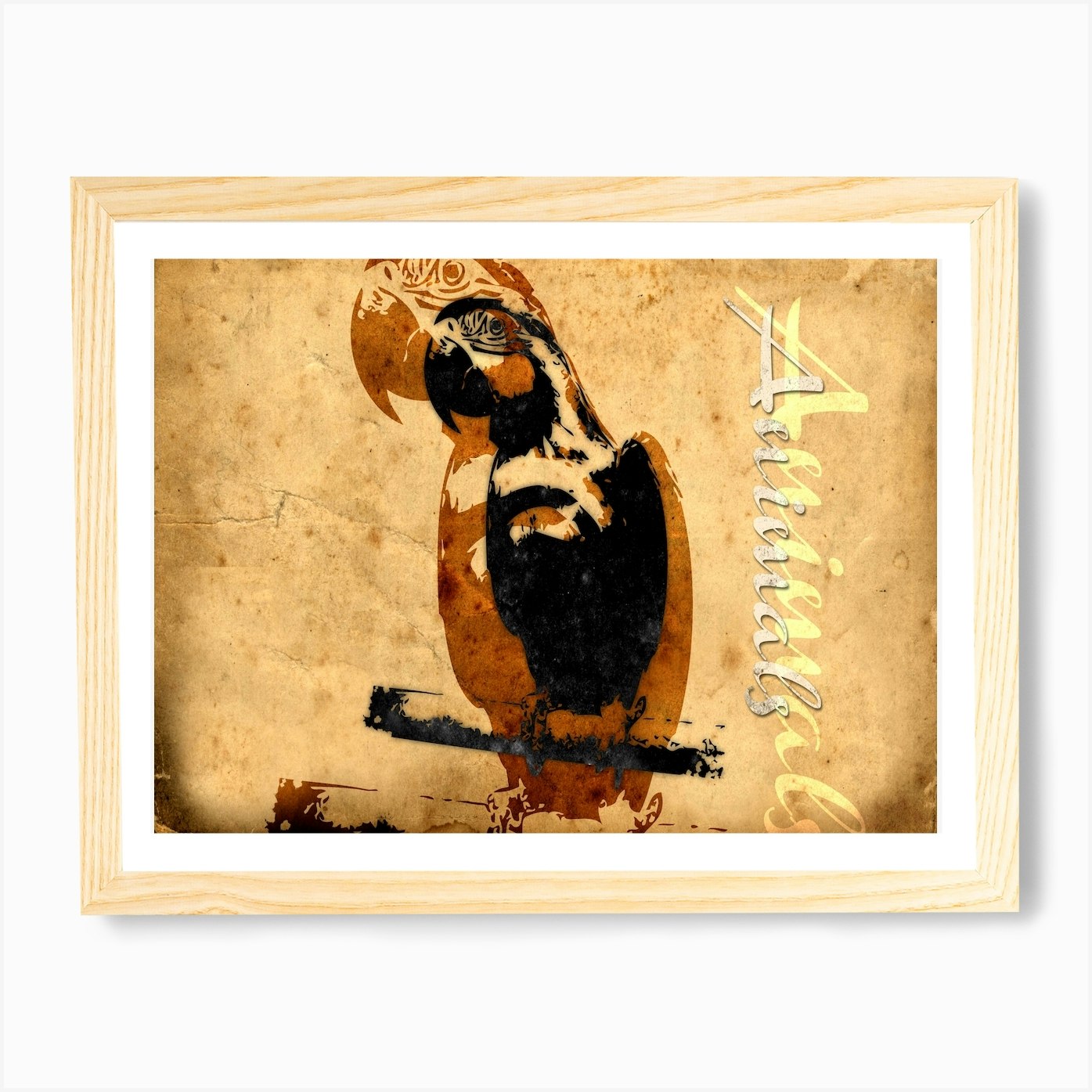This image showcases a stylized artwork of a parrot presented within a light wooden frame with a white border. The main subject is a black parrot with a notably long beak, depicted in an ink stamp style. Overlaid and slightly larger behind it is the same parrot, but in tan ink, creating an intricate layered effect. The backdrop resembles worn, vintage paper, enhancing the artistic feel. On the right side of the image, the word "animals" is written vertically in white cursive, accompanied by a larger yellow shadow mimicking the same text style. The overall presentation is one of rustic elegance, with the aged paper texture and untreated wood frame complementing the detailed and carefully layered parrot imagery.